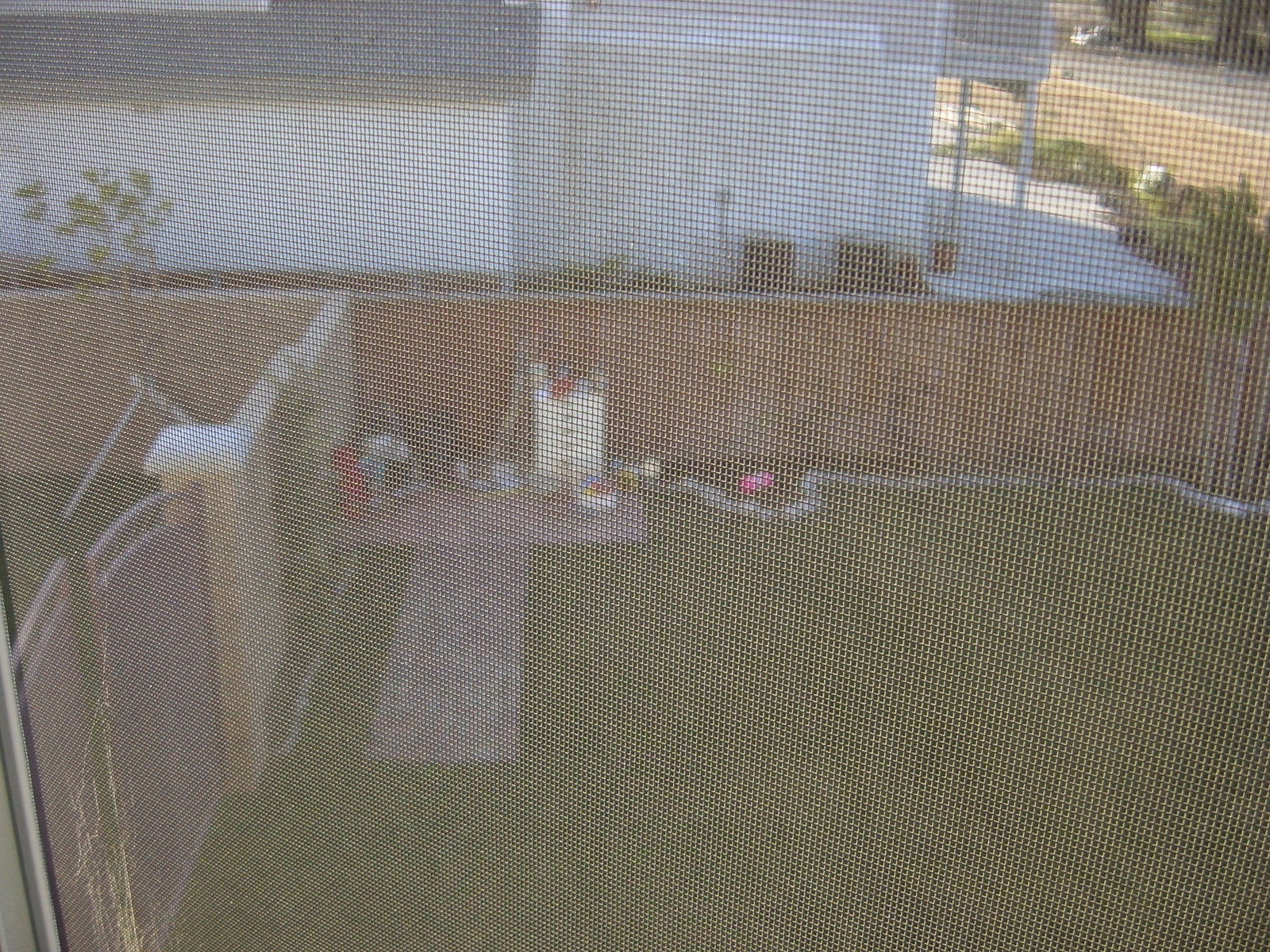This grainy photograph, taken through a window screen, captures a detailed view of a backyard scene. The image is divided horizontally, with the lower half showcasing a lush green lawn and the upper half revealing glimpses of a neighbor’s white house, complete with a balcony visible on the second story. A prominent feature in the backyard is a stone wall adorned with a decorative wooden gate featuring rounded tops, leading to a brick walkway that continues onto a brick patio. In the top left corner of the lawn, there is a children's play area, evidenced by a life-size dollhouse and a scattering of white and red toys. This area is bordered by a wooden fence that runs perpendicularly out from the stone wall, creating a distinct partition in the yard. Additionally, a stone border outlines a landscaped section in the right corner of the yard, while a road and some shrubbery are faintly visible in the top right of the image.